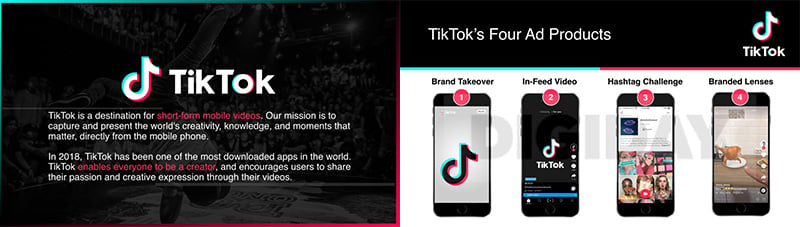This image, taken from a page about TikTok, prominently features a black background with faint, illustrative drawings subtly incorporated around the edges. On the left side of the image, there is a musical note depicted in blue, green, white, and red hues. Superimposed over this note, the word "TikTok" is displayed in bold white lettering.

Below the TikTok logo, a detailed mission statement can be seen: "TikTok is a destination for short-form mobile videos. Our mission is to capture and present the world's creativity, knowledge, and moments that matter directly from the mobile phone." 

Following a slight space, it continues: "In 2018, TikTok has been one of the most downloaded apps in the world. TikTok enables everyone to be a creator." Notably, the phrase "everyone to be a creator" is highlighted in red, while the remaining text is white. It concludes with, "and encourages users to share their passion and creative expression through their videos."

Towards the top of the image, the text "TikTok's Four Ad Products" is displayed, accompanied by four smartphones, each showcasing different aspects of TikTok's advertising options.